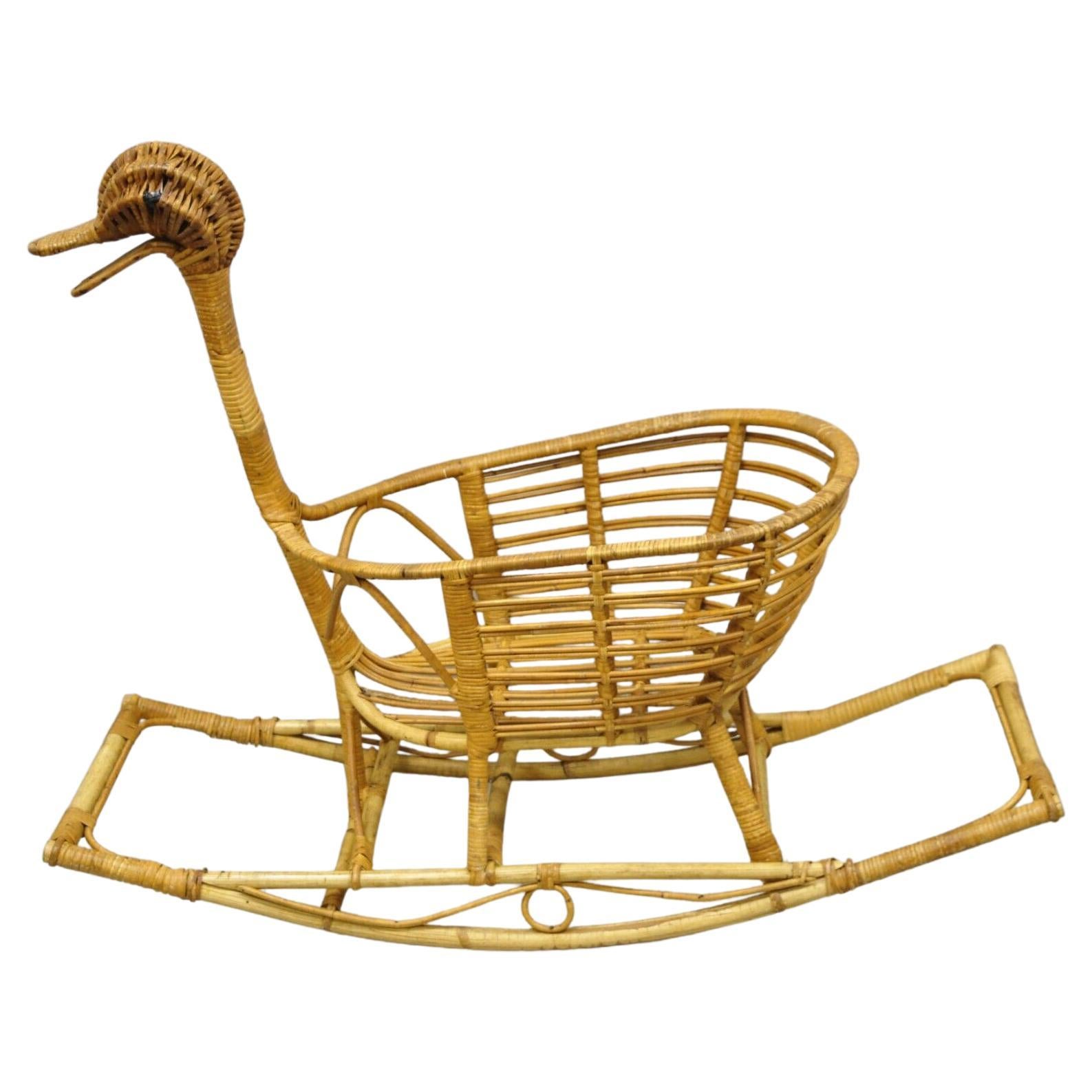The image shows a detailed photograph of a distinctive bassinet that doubles as an ornamental piece of furniture. Made from cane or bamboo sticks, this rocking bassinet features a central hollow shape designed to cradle a baby. The body of the bassinet is woven in a striped pattern, and it rests on a wooden curved base that allows for a soothing rocking motion. Notably, the bassinet is adorned with the head of a duck positioned to the left side, characterized by a darker brown color, an open beak, and a black, beady eye. The elegant yet functional design makes it both a practical crib and a charming decorative object.